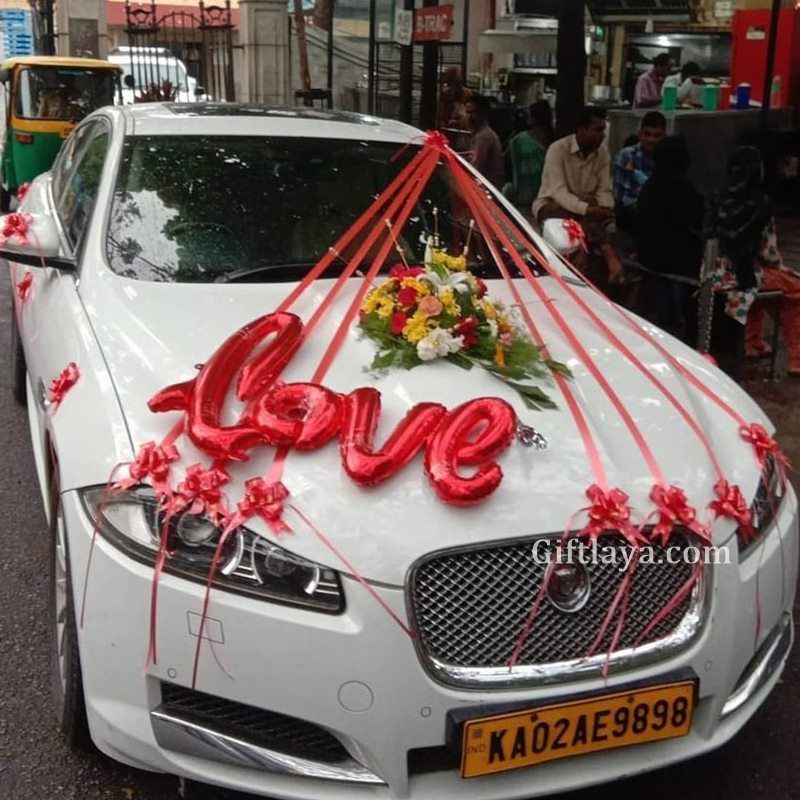The image showcases a brand-new white four-door car, adorned as a gift, parked outside an open-air restaurant. The car, facing the camera, has a sunroof and a distinctive chrome front grille with a centered chrome circle, and it sports a yellow license plate reading KA02AE9898. Decorated with festive elements, the car features seven red ribbons stretching from the top of the driver's side door across the front hood, each adorned with bows. Prominently displayed on the left side of the hood is a red balloon with the word "LOVE." A vibrant bouquet of flowers with green leaves, yellow, red, and white blooms sits on the car's roof. In the backdrop, diners are seated at tables, engaged in conversation, possibly hinting at the location being India. The name "giftleia.com" is subtly displayed in light gray on the right side of the image. Behind the car, a green vehicle and distant buildings are partially visible.